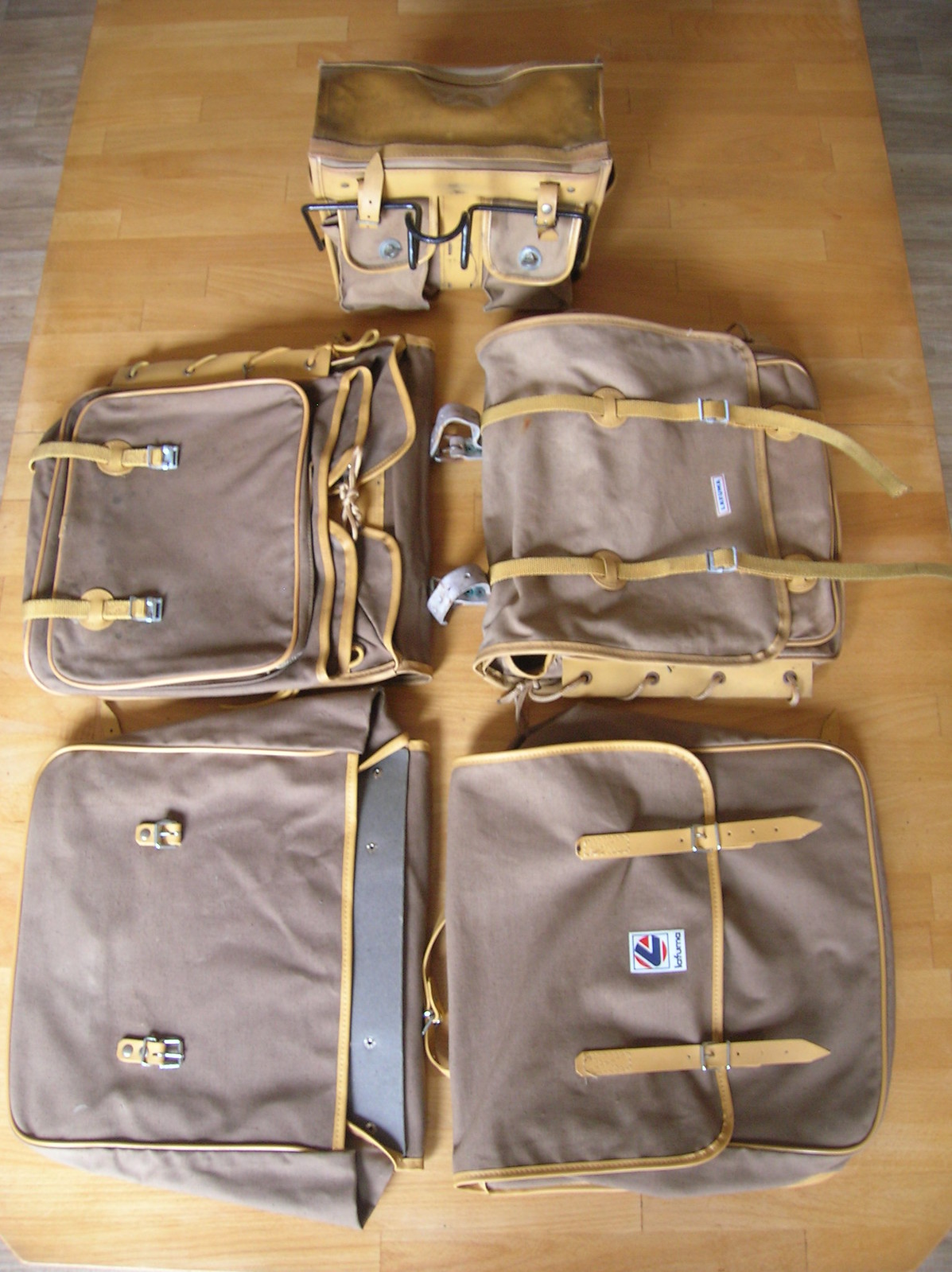The image shows a carefully arranged set of five bags on a light brown wooden table with a butcher block pattern. There are four U-shaped, dark grayish brown messenger-style bags with flat tops and light tan leather straps and borders. These bags are divided into two rows, each pair facing opposite directions. They feature white labels with a round logo consisting of a blue 'L' or arrow shape and red accents, indicating their brand. The front flaps of these bags are secured with leather straps and silver buckles. Positioned at the top center of the image is a tan square canvas bag distinguished by a complex metal hook mechanism on the front, similar to a lunchbox or handlebar bag for bicycles. This bag also has two front pockets with snap closures and a zip-around top, complete with a black metal frame. The entire setup suggests these satchels and saddlebags are likely designed for bicycle use, providing a practical yet stylish storage solution for riders.